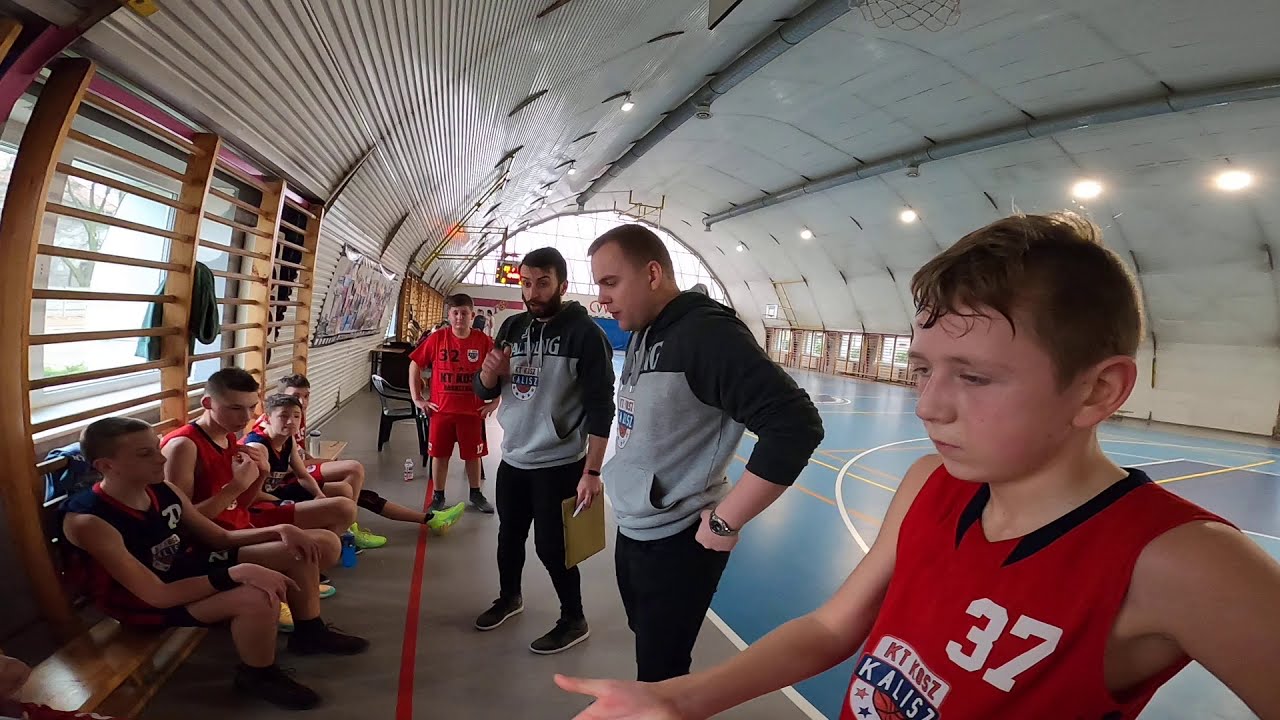The image depicts a boys' basketball team inside a large gymnasium with a distinctive domed ceiling, likely a Quonset hut. The center of the photo features two older men, presumably coaches, dressed in matching sweatshirts with black sleeves and gray bodies, along with black pants. One coach with a beard holds a clipboard. They appear to be addressing the team, which comprises six boys in red uniforms and one in black.

Four boys are seated on a wooden bench, attentively facing the coaches, while two others stand. The boy closest to the camera, who is sweating and has short dark hair, is wearing a distinctive red tank top with the number 37 and a logo that includes "K-T-K-O-S-Z" on a white box with a blue box below it that says "K-A-L-I-S". This suggests the team might be from Russia or Eastern Europe. The gymnasium features a smooth blue basketball court with white lines. Behind the team, large open windows are visible at the far end of the domed roof, contributing to the well-lit atmosphere.